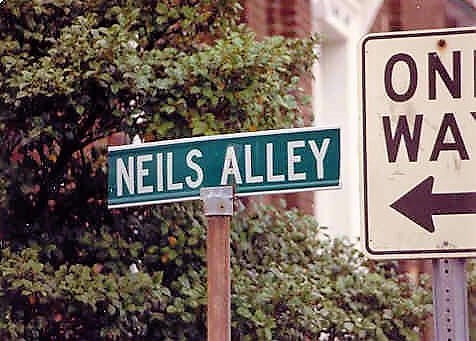The photograph captures a street scene prominently featuring a green street sign with white lettering that reads "Neal's Alley," mounted on a wooden pole. Adjacent to this, partially visible, is a black and white, square one-way street sign fixed on a metal pole, with an arrow pointing towards Neal's Alley, indicating that the alley is a one-way street. In the background, a tall tree with lush green leaves rises above the street sign, partially obscuring a towering red brick building that stands further back, adding depth and urban context to the scene.